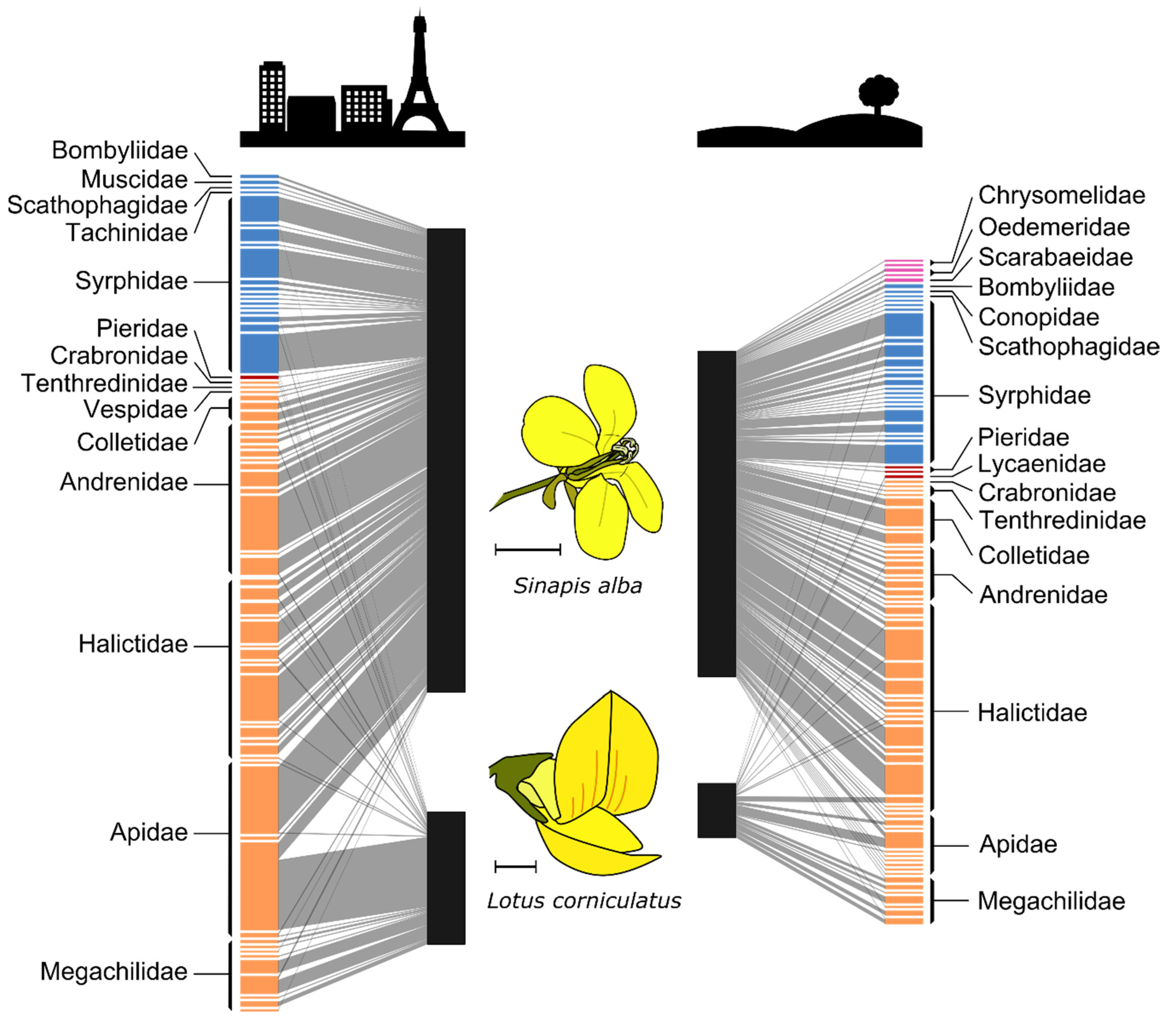The image depicts a detailed scientific diagram featuring various parts and nomenclatures related to flowers. Central to the image are two flowers with yellow petals labeled as *Sinapis alba* and *Lotus corniculatus.* Surrounding these flowers are intricate columns of black lines with numerous gray offshoots branching into blue, orange, and pink lines. These offshoots contain dozens of scientific names, such as *Bambilidae,* *Muscidae,* *Chrysomelidae,* and *Odimeridae,* representing different flower parts or related organisms. At the top, the diagram includes a black-and-white illustration of several city buildings, including a tower and a structure resembling the Eiffel Tower, positioned on the left. On the right, there's a drawing of a hill with a small tree. The arrangement of elements suggests a complex chart detailing the taxonomy or classification of the flowers and related species, enriched with vibrant colors including yellow, light yellow, black, gray, blue, orange, green, and olive green. The overall style is scientific and meticulous, highlighting the diversity and specific nomenclature in botany.